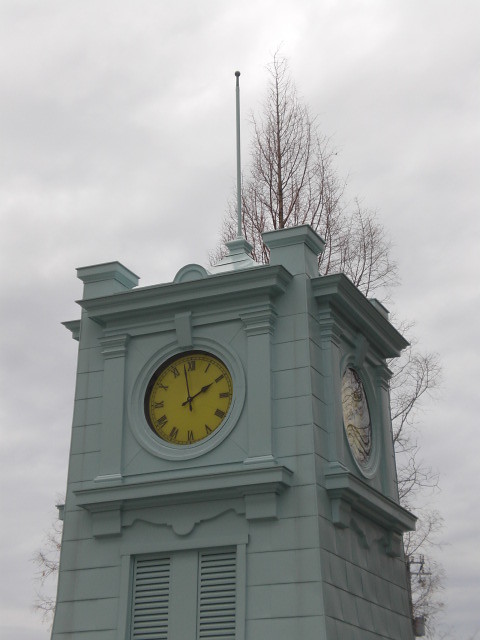Under a foreboding, cloudy gray sky that barely allows any sunlight to penetrate, the image prominently features an imposing clock tower in the foreground. The tower, with its grayish-green hue, stands tall and is topped with a roof that culminates in a square shape. Each side of the tower boasts round clocks shielded by yellow-tinted glass. Flanking the structure are two robust stone columns, lending an aura of strength and stability. The base of the tower appears to have what look like shutters, enhancing its architectural detail. To the right, another clock is visible, both clocks resting above protruding ledges. Behind the tower, a row of trees adds a natural contrast to the somber scene. At the pinnacle of the tower, a flagpole stretches upward, completing the tower's stoic presence against the dreary backdrop.